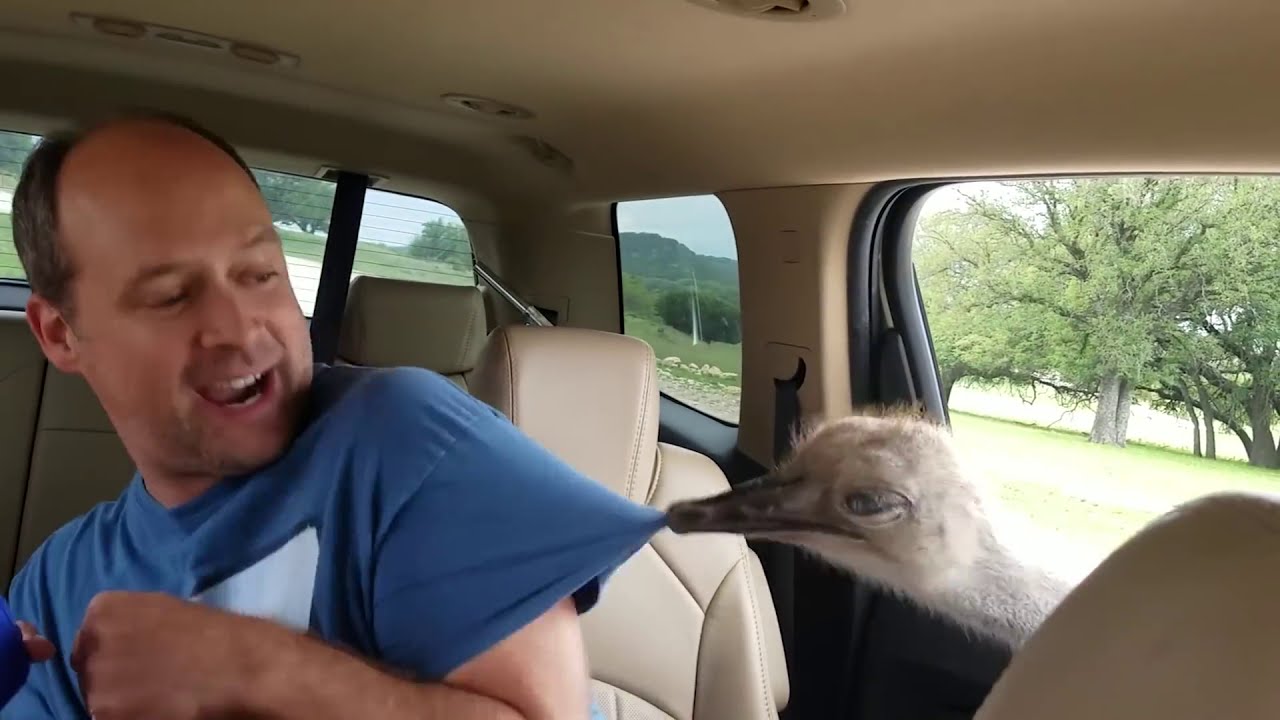In this vibrant daytime scene, a man with a receding hairline and brown hair, dressed in a blue shirt featuring a white patch on the chest, sits inside a beige interior car. He is leaning to the left, his mouth open and teeth visible, displaying a look of mild surprise as an ostrich pokes its gray head through the car window. The ostrich, with its darker gray beak, tugs playfully on the man's sleeve. The interior of the car is composed of cream-colored leather seats and a matching ceiling. Outside the car window, a picturesque landscape unfolds with large green trees, a lake, and distant mountains under a hazy white sky.